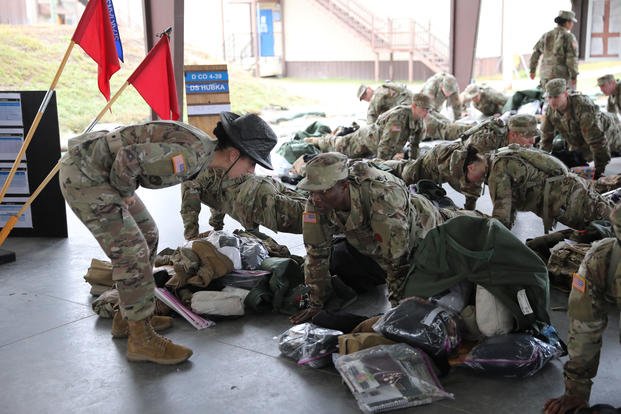In this photograph, we see a group of approximately 20 army recruits performing push-ups on a grey ground, indicative of a rigorous training session at what appears to be an army boot camp or barracks. The recruits, dressed in brown and green camouflage uniforms, are in the up position of their push-ups, indicating the intensity and discipline of their training. In the foreground, on the left side, a female drill sergeant stands in a hunched position, seemingly motivating and commanding the recruits as she stares intently at one of them. She is also clad in army attire. To her left, two red flags are affixed to poles. Scattered on the ground around the recruits are various military gear and personal belongings, including large duffel bags that have spilled their contents, suggesting the recruits have recently arrived and are undergoing initial training scrutiny. The background reveals a building with visible stairs, adding to the environment's authenticity as a military training facility.